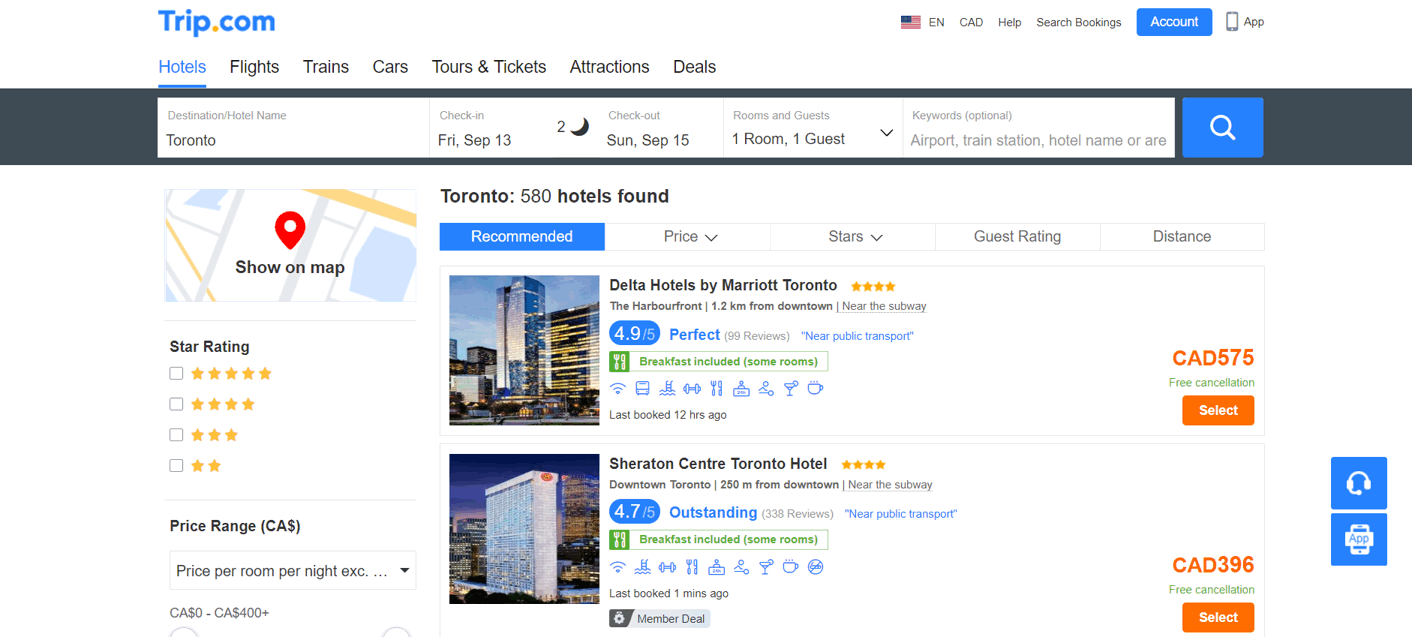This is a detailed screenshot of the Tripp.com website. At the top left corner, the Tripp.com logo is prominently displayed, with 'Tripp' in blue and the dot in orange. On the top right side of the header, there are several options: 'EN' (representing the English language), an American flag icon, 'CAD' (indicating the currency), 'Help', 'Search Bookings', 'Account' (shown as a solid blue button with white text), and 'App'. All other text in this section is black.

Below the header is a navigation bar with buttons for different services: 'Hotels', 'Flights', 'Trains', 'Cars', 'Tours & Tickets', 'Attractions', and 'Deals'. The 'Hotels' button is highlighted in blue and underlined, signifying the currently selected category.

Underneath the navigation bar, search fields are presented for booking a hotel. These fields include:
- Destination/Hotel Name: 'Toronto'
- Check-in Date: 'Friday, September 13'
- Check-out Date: 'Sunday, September 15'
- Rooms and Guests: 'One room, one guest'
- Keywords (optional): 'Airport, train station, hotel name, ORR'

A blue 'Search' button is available for users to initiate the search with the specified criteria.